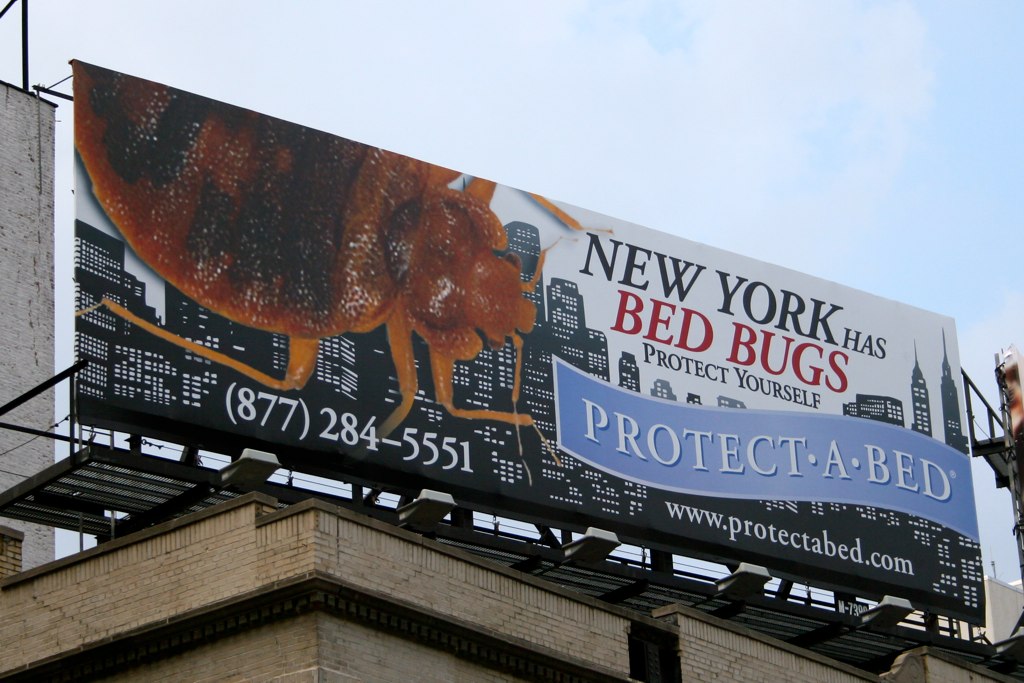A large billboard stands prominently atop a rooftop in the city, catching the eye with its striking imagery and clear message. The billboard, approximately twice as wide as it is tall, features a silhouette of the iconic New York City skyline under a relatively clear blue sky, dotted with small patches of clouds. Dominating the scene, a giant, blown-up depiction of a bedbug crawls ominously over the buildings, symbolizing a widespread concern. The text on the billboard reads, "New York has bedbugs. Protect yourself, protect a bed," followed by the website, "protectabed.com" and a phone number for more information. The clear and attention-grabbing design conveys a sense of urgency, urging passersby to take action against the bedbug issue.